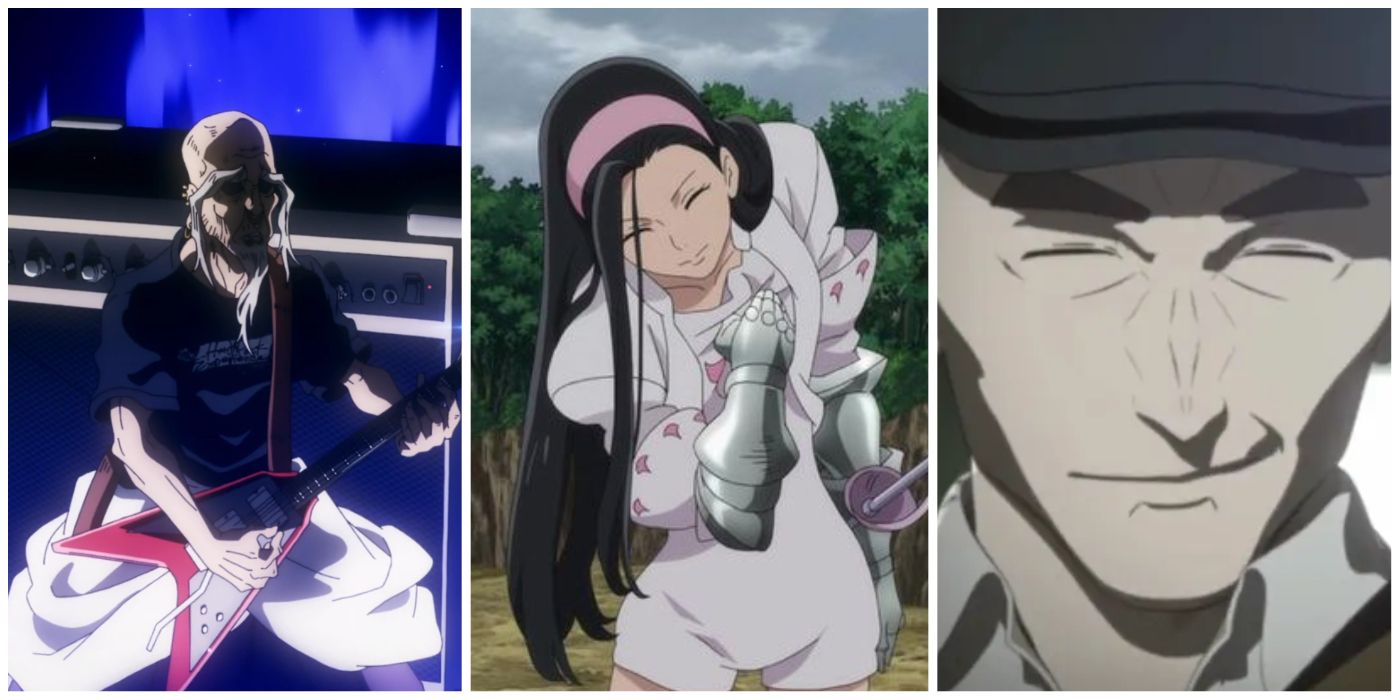This detailed anime-style image features three distinct illustrations side by side. On the far left, there's a zoomed-in depiction of a man playing a red, V-shaped electric guitar. The man, who seems to be performing on a concert stage, is wearing puffy white pants and a black shirt adorned with some writing. Despite the shadows on his face, his intense expression is noticeable. He has long white eyebrows, a white goatee, and appears to be balding. Behind him, an amplifier or switchboard is visible, with a blue glistening glow in the background.

In the center, a woman is illustrated with a striking sense of emotion. She has long, flowing black hair that extends to her waist, adorned with a pinkish-purplish headband. Her eyes are closed as she leans her head down, her right arm clutched to her chest with what appears to be a silver, metal-like glove, while her left arm is by her side, suggesting she might be holding a fencing foil. Her outfit is a pink romper with cap sleeves, harmonizing with the headband. The background behind her features greenery, providing a contrasting serene environment.

On the far right, another man is portrayed with a scrunched up, squinting face, rendered in beige tones. He is wearing a dark gray hat and the collar of his gray shirt is visible. His expression is intense, and the simplicity of the sketch emphasizes his focused gaze. Together, these three captivatingly detailed images create a dynamic and emotionally engaging triptych.